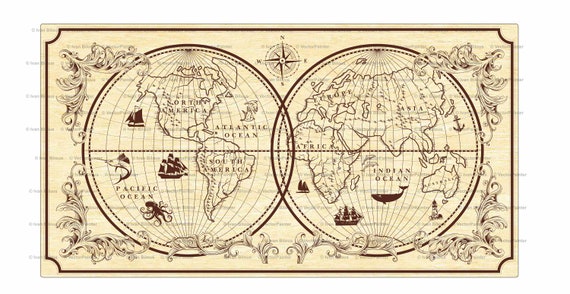This detailed, rectangular image features a vintage-style map on a cream-colored background with dark brown accents. The map is divided into two slightly overlapping circles, filled with detailed illustrations. The left circle contains North America, South America, the Atlantic Ocean, and the Pacific Ocean, while the right circle displays Europe, Africa, Asia, Australia, and the Indian Ocean. Both circles include intricate sea creatures such as whales and octopuses, along with sailing boats, emphasizing the aged, ornate style of the piece. A prominent compass is placed at the top center, and the border is adorned with decorative filigree designs, enhancing the historical and hand-drawn appearance typical of the 1800s or early 1900s cartographic art. A horizontal dotted brown line runs across the middle of the map, further adding to its antique aesthetic.